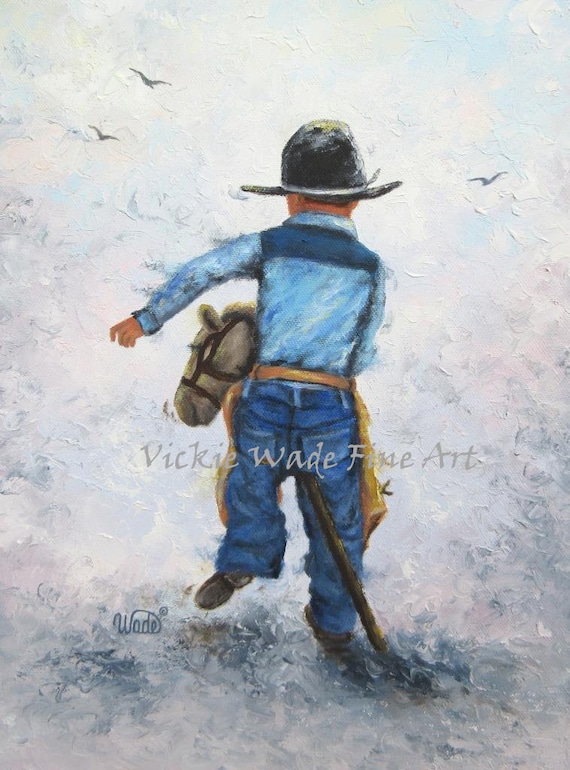This is a painting by Vicky Wade Fine Art, identifiable by a watermark in the image. The artwork portrays a small boy dressed in a Western cowboy outfit, seen from behind. He is wearing a black cowboy hat, a Western-style collared shirt that is two shades of blue—light blue with a dark blue top—and blue jeans. Complementing his attire, he has a brown, harness-like belt that hangs at his sides, and he is wearing brown shoes.

The boy, whose face is not visible, is joyfully riding a wooden stick horse, complete with a horse head at the end, embodying the spirit of imaginative play. The stick horse's head is discernible to the left of the boy. The background of the image is textured and predominantly gray, casting a shadow underneath him, with three birds—likely seagulls—flying in a sky that mingles white and blue hues. The uniqueness of the painting is accentuated by what appear to be brushstrokes, suggestive of acrylic or watercolor techniques. Below the boy’s left foot, the word "Wade" is inscribed, possibly as a signature or watermark.